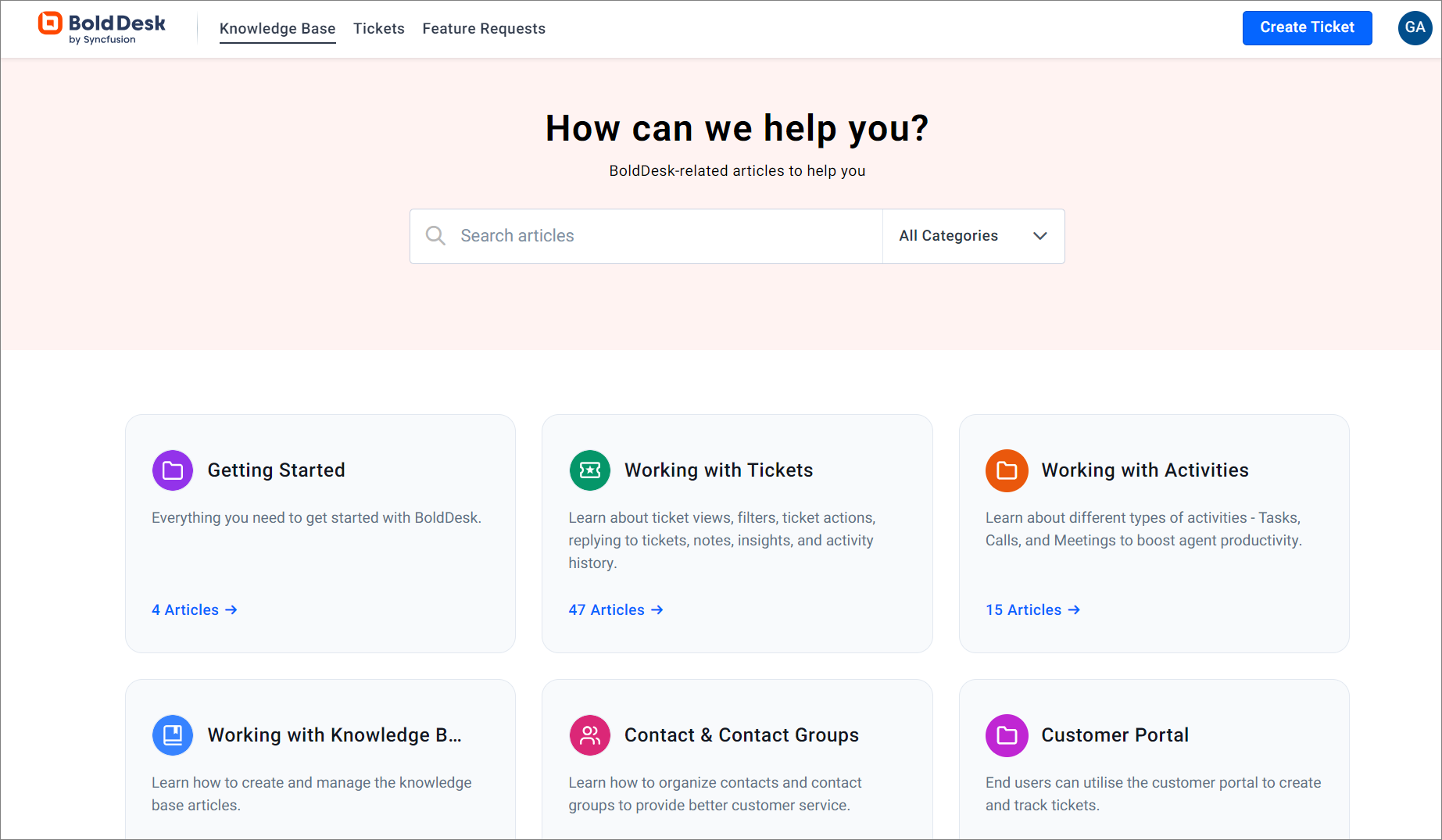This is a screenshot of the BoldDesk website homepage. In the top left corner, the website name "BoldDesk" is prominently displayed. Adjacent to this, there are several navigation tabs: "Knowledge Base," "Tickets," and "Feature Requests." The "Knowledge Base" tab is highlighted with a black underline, indicating it is the currently active section.

In the top right corner, there is a blue button labeled "Create Ticket" in white text, inviting users to initiate a support request. Centrally positioned at the top, a large black text headline asks, "How can we help you?" Immediately below this, there is a search bar allowing users to search all categories, with options for filtering searches to specific categories.

Further down the page, there are various sections providing overviews and helpful resources. On the top left, a section titled "Getting Started" features a purple folder icon and a description, "Everything you need to get started with BoldDesk." Additional sections below include "Working with Tickets," "Working with Activities," and "Customer Portal," each providing more detailed information about different aspects of the website. Overall, the homepage serves as a comprehensive and user-friendly guide to navigating the BoldDesk platform.